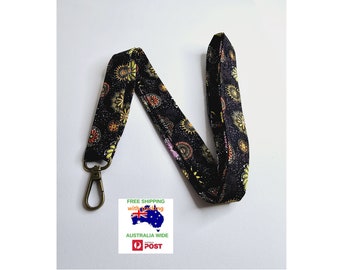This image features a black velvet lanyard adorned with a pattern of yellow medallions and variously colored flowers—including shades of red, pink, and yellow—printed along its length. The lanyard appears wider than usual and terminates in a dark brown, carabiner-like clasp, useful for attaching a name badge or keys. It rests on a white background. In the lower part of the image, there's a text box with a free shipping offer. The text reads "free shipping with tracking" in green and orange fonts. Beside the text, there's a blue shape of the Australian landmass with the Australian flag's colors and the phrase "Australia-wide" in green, followed by the word "post" in red, accompanied by a red symbol.